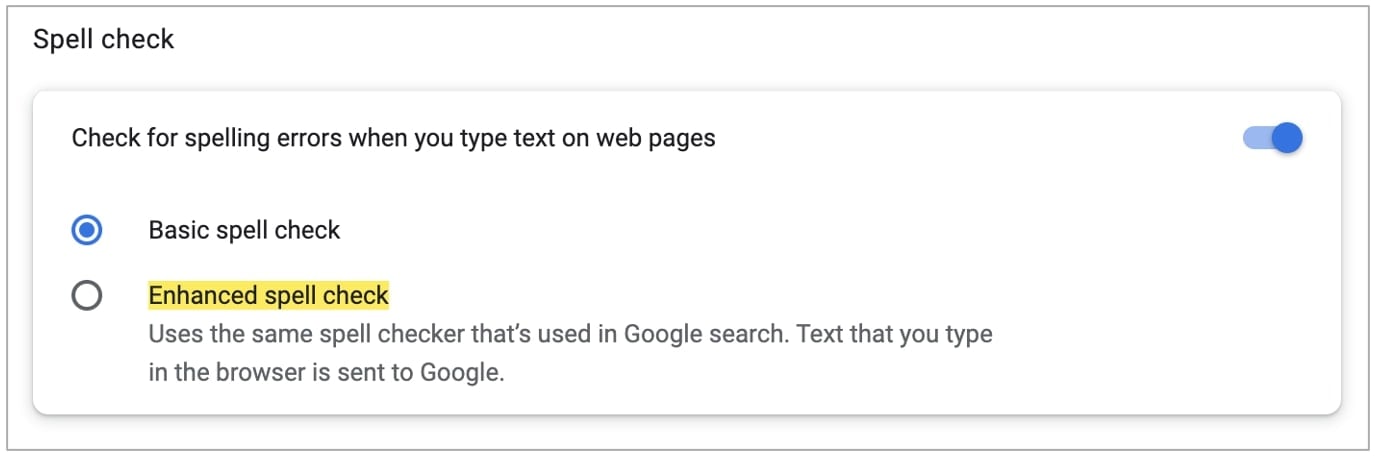In the screenshot, which features a predominantly white background, there is a gray-outlined rectangle. In the upper left corner, black text reads "Spell Check." Beneath this is another white rectangle containing bold black text that states, "Check for spelling errors when you type text on webpages." To the right of this text, there is a blue toggle switch indicating that the option is turned on.

Below the "Basic Spell Check" section, there is a circle on the left marked in blue. Underneath this section, the heading "Enhanced Spell Check" appears in bold and is highlighted in yellow. Next to this heading, there is a gray circle. Beneath this, the text reads, "Uses the same spell checker that's used in Google search. Text that you type in the browser is sent to Google."